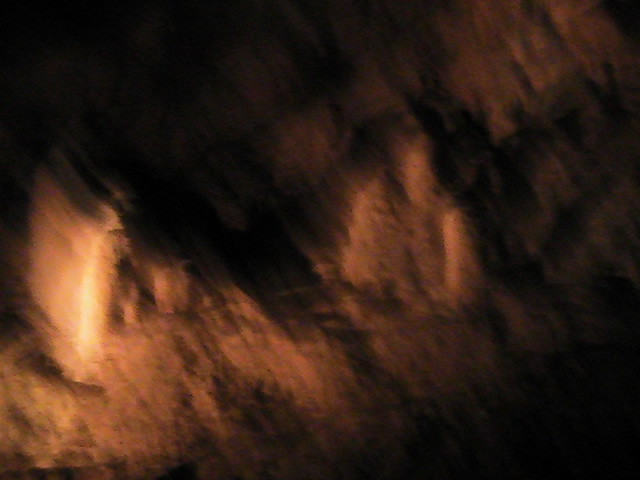This is a very blurry and dark image that seems to be a photograph taken in a dimly lit area. The overall coloration includes shades of black, brown, beige, and reddish-brown, giving the visual impression of an ancient, rocky environment similar to the inside of a cave. The photograph features jagged rocks or possibly the tops of trees, with the blurs stretching and angled to the left. A square object is discernible on the left side of the image, from where a light source is casting a glow over the middle section. The bottom right and top left corners are completely black, adding to the image's mystery. In the center, there are two arched areas, with a tiny object inside the left arch, and the light contrasts intermittently suggest some moonlight casting flashes over the scene. The blurriness and indistinct appearance of shadows and shapes make the visual experience surreal and enigmatic.